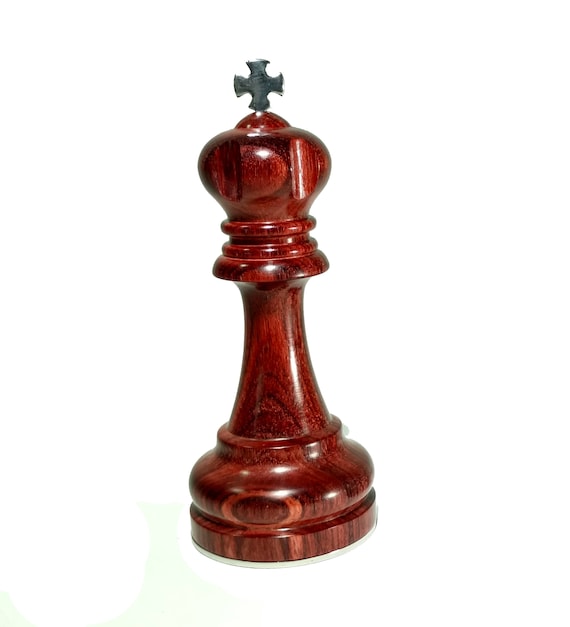The image showcases a single chess piece resembling the king, crafted from dark brown wood with a distinctive red stain that highlights the wood's grain. It has a glossy finish, with noticeable sheen and light reflections that accentuate its smooth surface. The piece features a rounded bottom, grooves carved into the wood, and a distinctive globular top. At the very top, there's a dark gray, cross-like metal piece, indicating the figure's status as a king. The chess piece, which appears handmade, is photographed against a plain white background, emphasizing its detailed craftsmanship and rich color.